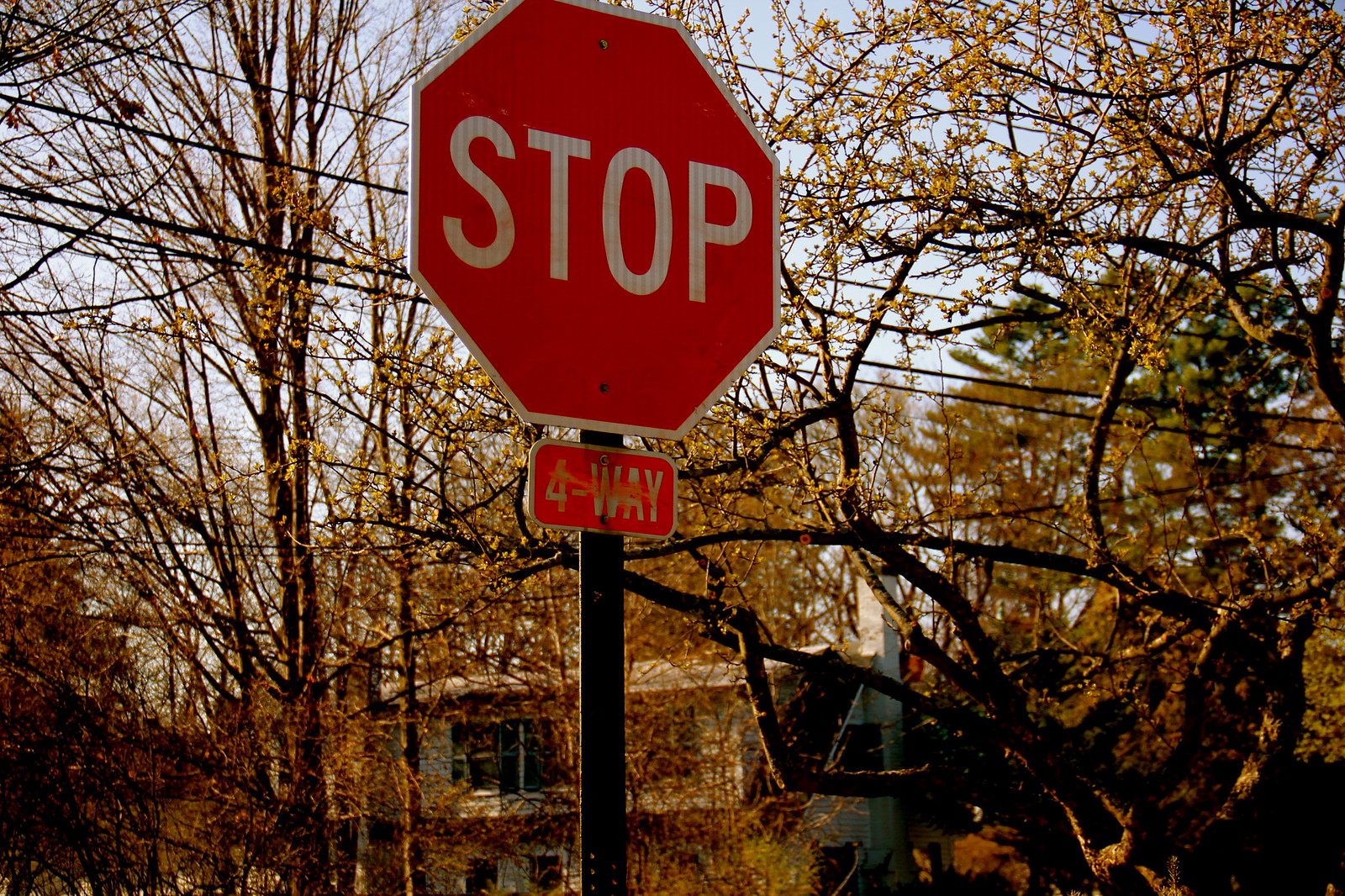The image is a detailed close-up of a bright red stop sign at the center, with "STOP" written in bold white letters. Attached below it, a smaller red rectangular sign reads "FOUR-WAY." The background reveals a neighborhood scene characterized by its autumnal setting. Dense trees with thin trunks and numerous branches sport small, vibrant yellowish-brown leaves, illuminated by the light. Interspersed among the foliage, visible in the lower center behind the stop sign, is a partially obscured house, distinguishable by its white chimney on the right side. The house's overall color remains indeterminate due to the dense foliage. Overhead, several electric power lines span from left to right, adding to the intricate backdrop. The trees are somewhat bare, suggesting a transitional season with some leaves still clinging to the branches. The scene has a somewhat overgrown and neglected feel, with no people, animals, or vehicles present, emphasizing the stop sign as the image's focal point.